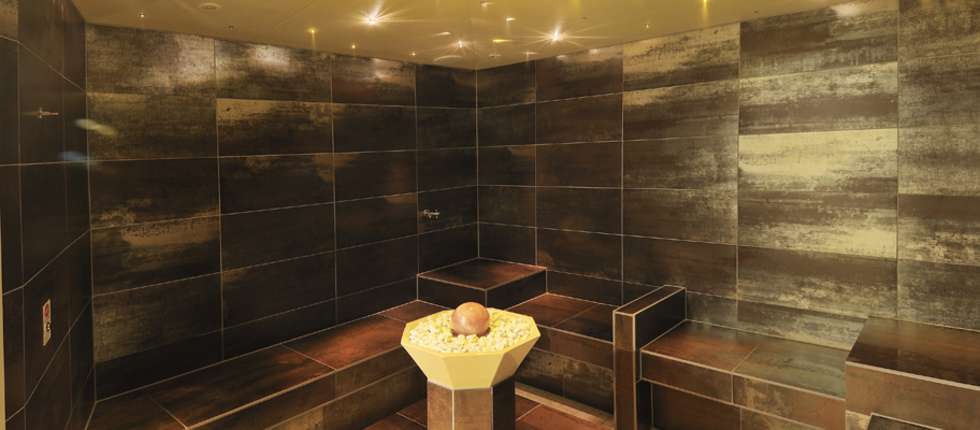The image captures an interior setting that resembles a luxurious sauna or steam room, likely found in a high-end spa or hotel. The room exudes sophistication with its dark brown, almost chocolate-colored walls and matching seating, all crafted from the same material. The walls and seating have sharp, angular edges, characterized by square and rectangular shapes without any curves. The surfaces reveal intricate textures, possibly of marble or ceramic, featuring subtle rust-like streaks and white inclusions. The ceiling stands out with its pristine white, polished marble-like finish and enhanced by elegant LED lighting.

At the room's center is a focal point: an octagonal stand holding a white bowl filled with small white stones, crowned by a smooth, round ball resembling a peach in a delicate pinkish hue. An off-center switch is also visible on the left side of the image. The color palette of the room includes rich browns, tans, blacks, whites, and peach-pink, contributing to its opulent and serene atmosphere.